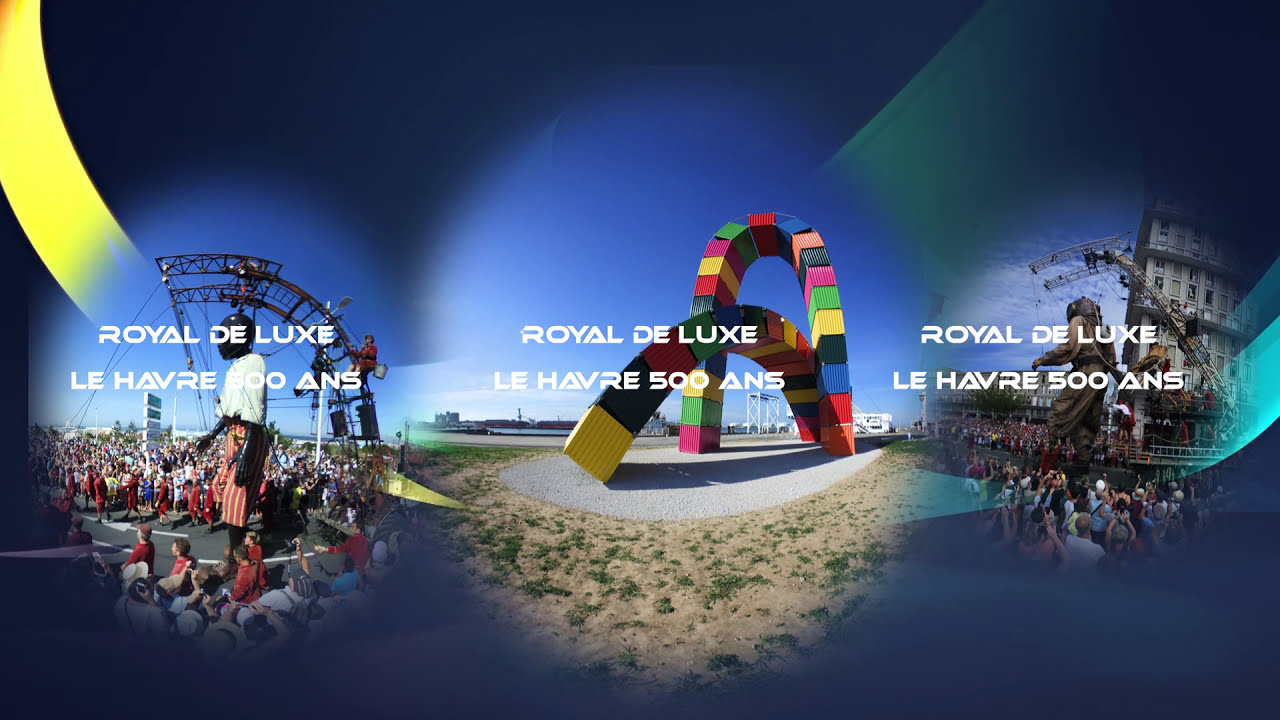The image depicts a vibrant outdoor scene featuring three main elements, each adorned with the text "Royal Deluxe Le Havre 500 ANS" in white. On the left, there is a circular image of a giant puppet dressed in a white shirt and red pants with white pinstripes, towering above a crowd of people. In the center, a colorful sculpture composed of interlocking rainbow blocks in pink, yellow, green, black, and red stands on a concrete paved area, surrounded by patches of green grass and sandy dirt. To the right, another circular image showcases a different giant puppet, held up by a mechanical grid structure, amidst a crowd of people with cameras, near a building. A bright yellow ribbon-like stripe starts from the top left corner, weaving through the dark blue background, enhancing the dynamic composition of this picturesque advertisement or postcard-like photo.